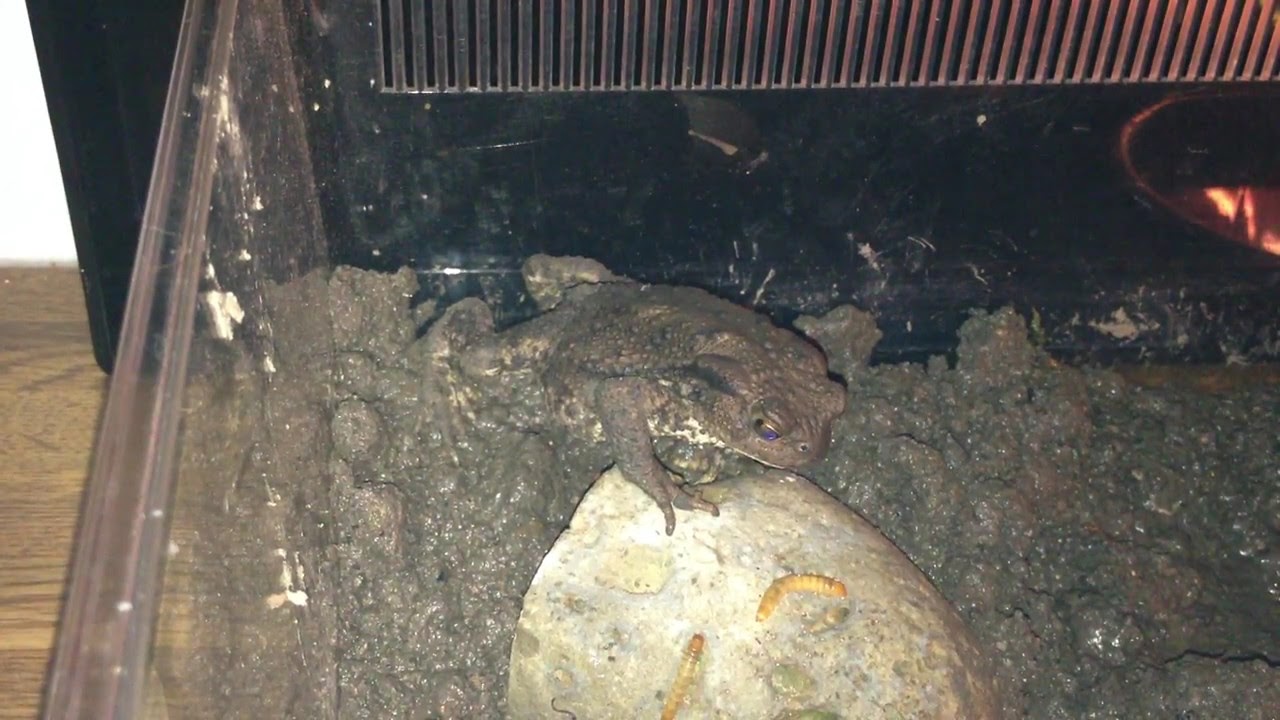The image captures an overhead view inside a cozy living room, focusing on an aquarium housing a brown toad perched on a gray rock. The toad, encased in a muddy, damp environment, has one arm resting casually on the rock while eyeing two mealworms, which it appears ready to eat. Surrounding the toad is a terrain laden with dirt and mud, giving a distinctly soggy impression. Behind the toad is a black radiator with a silver grate, adding a touch of household backdrop. A faint orange light shines onto the gray rock from the upper right corner, casting a warm glow. White markings are visible on the left wall of the aquarium, contrasting against the overall earthy tones. The aquarium rests on a light brown, hardwood floor, enhancing the homely setting.